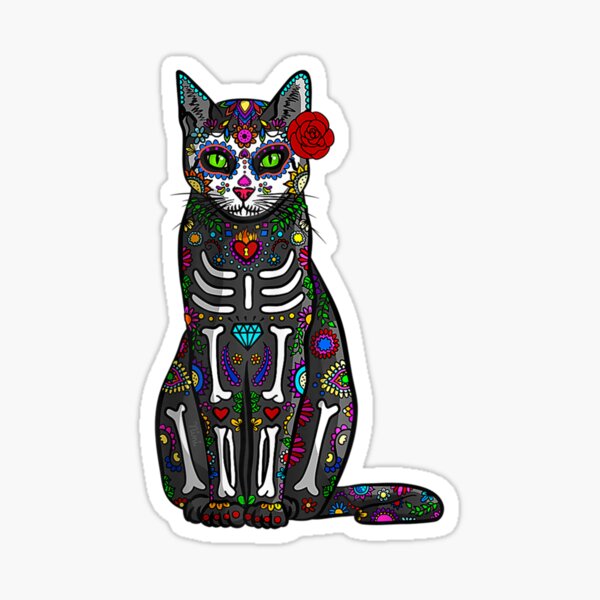This detailed image depicts a vibrant and colorful Day of the Dead cat sticker set against an off-white or beige rectangular background that is taller than it is wide. The cat is adorned with intricate designs and vivid colors reminiscent of the Mexican Day of the Dead celebration. The cat sits on all fours, predominantly black with a white face and striking green eyes. A prominent red rose is situated behind its left ear (the right side of the image). Highlighting its skeletal theme, white bones are artistically drawn throughout its body, accompanied by a red heart and a blue diamond on its chest area. The cat's decoration features a multitude of colors, including white, blue, gray, red, green, yellow, purple, pink, and orange, creating an eye-catching and vivid aesthetic. The entire image has a white border, contributing to a sticker-like appearance.